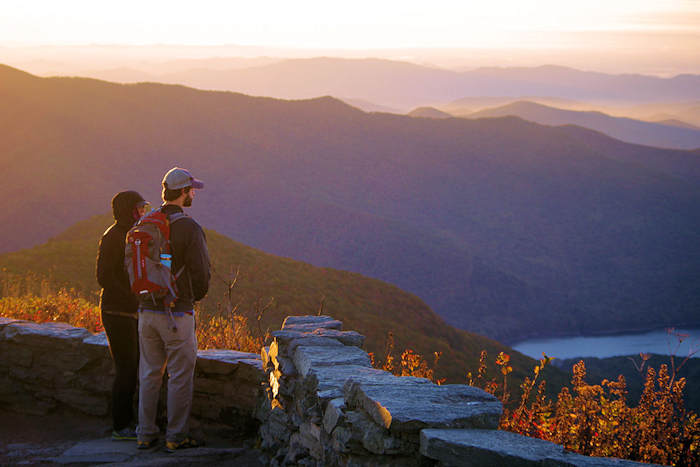In the photograph taken during sunrise or sunset, two people stand with their backs to the camera on a man-made rock structure, overlooking a vast valley. The person on the left is a man dressed in tan pants, a black long-sleeve jacket, and a gray hat, carrying a red and gray backpack. The individual beside him is dressed entirely in black, including a tracksuit with their hood up, making it difficult to discern their gender. They stand on a rocky lookout point with a two-foot stone fence, which extends up a smaller elevation against a backdrop of large green mountains to the left. The panorama before them features a river winding through the valley and lush trees in vivid autumn colors—reds, oranges, and yellows—illuminated by the golden light of the setting or rising sun.